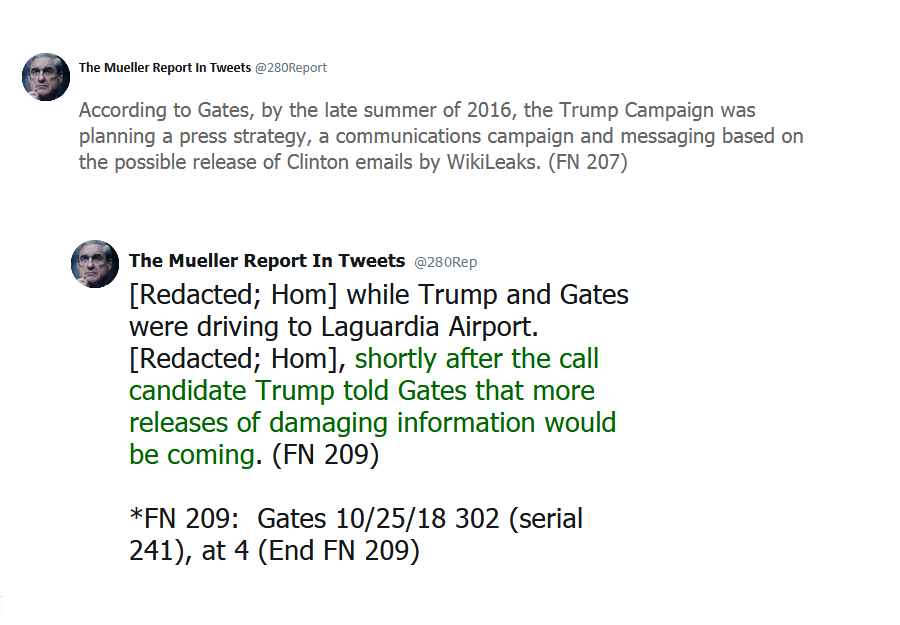This detailed caption summarizes an image of a Twitter post from the account "The Mueller Report in Tweets (@280Report)." The screenshot shows the older man’s profile picture in a circular frame and illustrates two tweets. The first tweet states, "According to Gates, by the late summer of 2016, the Trump campaign was planning a press strategy, a communications campaign, and messaging based on the possible release of Clinton emails by WikiLeaks (FN-207)." The second tweet, a reply from the same account, includes some redacted text and reads, "While Trump and Gates were driving to LaGuardia Airport [redacted], shortly after the call, candidate Trump told Gates that more releases of damaging information would be coming (FN-209).” Additional details note that FN-209 references Gates’ testimony dated 10/25/18, Serial 241 at 4. The text in the tweets varies in color, with some parts in black and others in green.